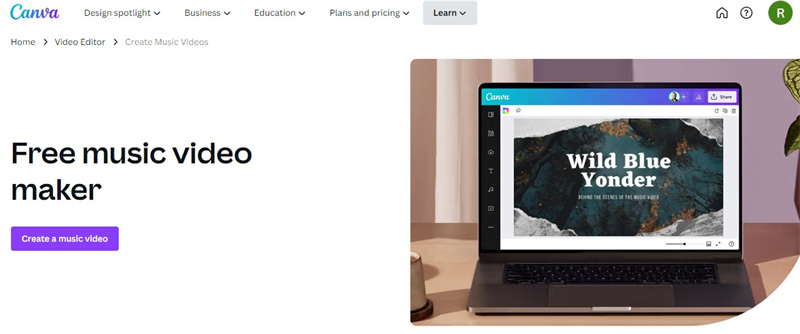This detailed caption describes an image from a company called Canva, showcasing their "Design Spotlight" interface for business education plans and pricing. At the top of the interface, "Design Spotlight" is boldly displayed. Beneath it, sections labeled "Business," "Education," and "Plans and Pricing" are prominently featured. A drop-down menu for "Learn," positioned in a gray rectangle, is visible alongside top navigation buttons for "Home" and "Question." A notable icon, a white "R" encased in a green circle, catches the eye.

Below this, on the left side, a navigation path starts with "Home," followed by an arrow leading to "Video Editor," and another arrow pointing to "Music." The path leads to the highlighted section, "Create Music Videos." Further down, in larger black print, the text reads "Free Music Video Maker," emphasizing the no-cost offer. Directly beneath this, a purple button with white text invites users to "Create a Music Video."

Adjacent to this textual information, the image includes a photograph of an open laptop displaying the Canva interface. The screen shows a mountainous background image with the text "Wild Blue Yonder" overlaid in white. This combination of text and visuals effectively communicates the functionality and attractive design capabilities provided by Canva for music video creation.